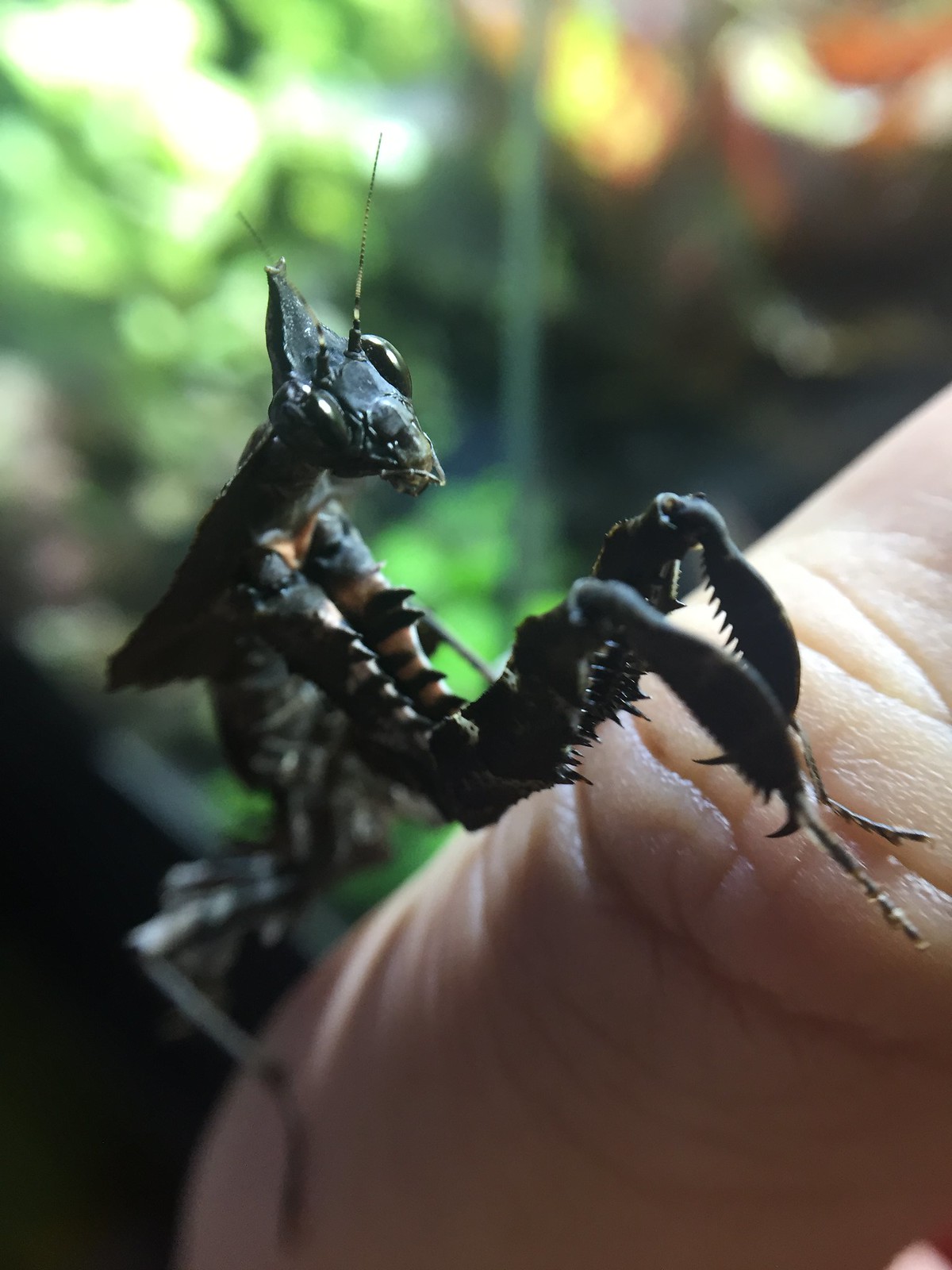The photograph captures a highly detailed and enlarged view of a black insect perched on a person's finger. The insect features two prominent, hook-like arms on its front abdomen, edged with yellow stripes and ending in sharp pointed hooks adorned with multiple spikes, resembling crab legs capable of crunching a walnut. The insect's head is diamond-shaped with large, oval, bulbous eyes and two long, striped yellow and black antennae emerging from the center. While the rest of its body remains blurred and out of focus, more additional legs can be seen, all positioned on the finger. The background shows an out-of-focus vegetation scene, adding to the natural setting of the image.